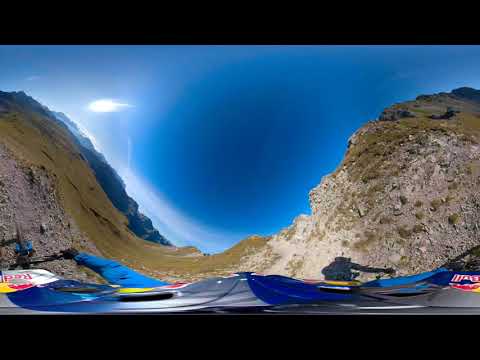This distorted image, possibly captured with a 360-degree camera, shows an outdoor scene featuring rolling, rocky hills with patches of moss and greenery. Dominating the foreground are what appear to be elongated and stretched jet skis in blue, yellow, and white, marked with red lettering. A notable shadow cast on the rocky hills in the background hints at a person who could be riding a jet ski. The terrain includes a mix of light gray stone, dirt, and sparse grassy patches, creating a rugged landscape. The blue and silver Red Bull helmet of a mountain biker, visible at the lower portion of the image, is flattened and skewed horizontally from left to right, adding to the warped effect. The sky above is blue with a noticeable glare on the left side, suggesting bright daylight conditions. This peculiar composition, with hints of colored material and a shallow valley between the peaks, creates an intriguing and surreal snapshot of a mountainous outdoor adventure.